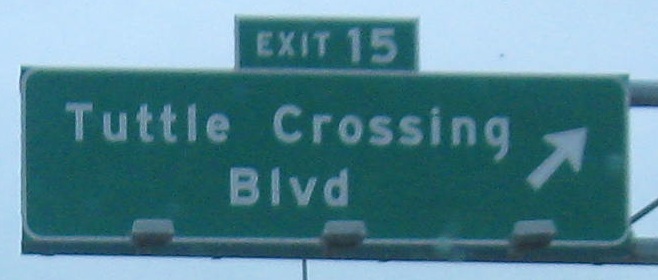The photograph captures a highway exit sign for "EXIT 15" and "TUTTLE CROSSING BOULEVARD." The sign is predominantly green with white text and a white border. The smaller "EXIT 15" sign sits above the larger "TUTTLE CROSSING BOULEVARD" sign, which includes an arrow pointing diagonally up and to the right, indicating the direction of the exit. The sign is supported by a metal frame with some parts and rods visible. The background shows a misty, cloudy sky that is light blue, suggesting the picture was taken during the day but under dull and possibly wet conditions. The scene includes three light housings on the lower half of the sign, and the image appears a bit grainy and out of focus. No other details or text are visible in the photograph.